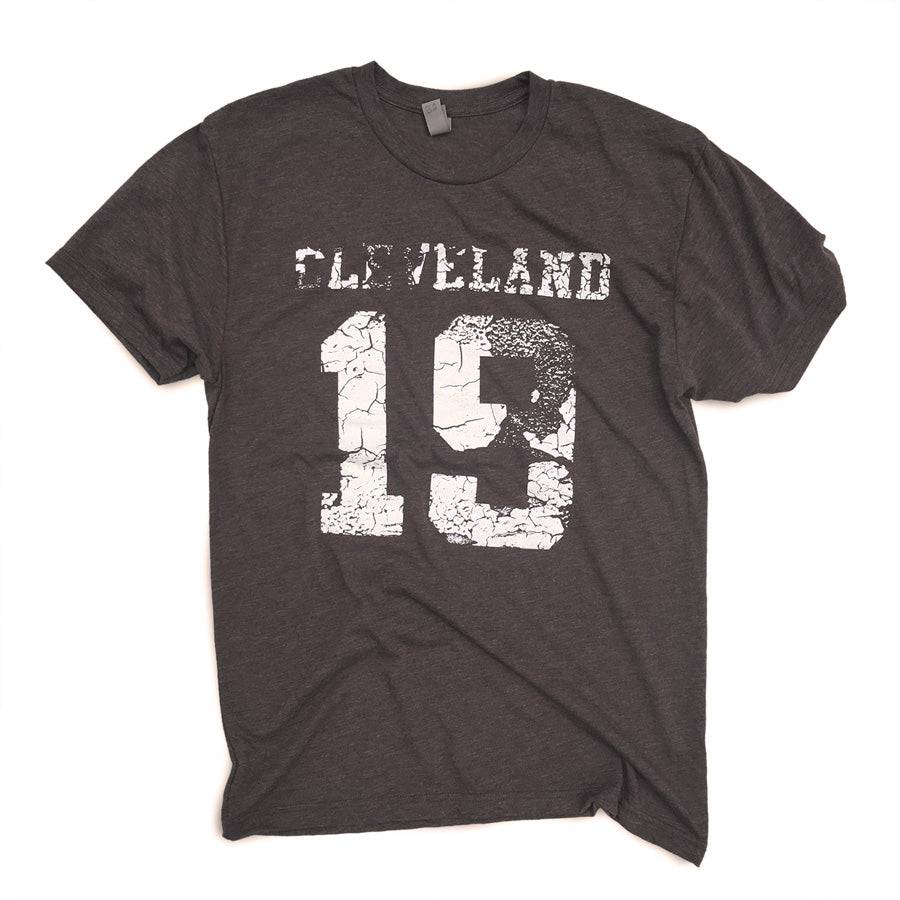This image depicts a well-worn, short-sleeved, charcoal gray t-shirt laid out on a white background. The shirt features a crew neck style with a gray tag that is flipped up at the back of the neckline. Across the chest in large, worn white letters, it says "CLEVELAND," with significant cracking and fading, especially noticeable on the bottom of the 'C,' the 'E,' and the left side of the 'V.' Below that, near the stomach area, the number "19" is displayed, similarly distressed with the '9' almost completely worn away. The t-shirt has a textured look with some stylistic wrinkles, especially noticeable in the upper right and lower sections. Despite its tattered appearance, which shows signs of frequent washing and wear, the shirt retains a sense of comfort, indicative of a beloved and well-used garment.